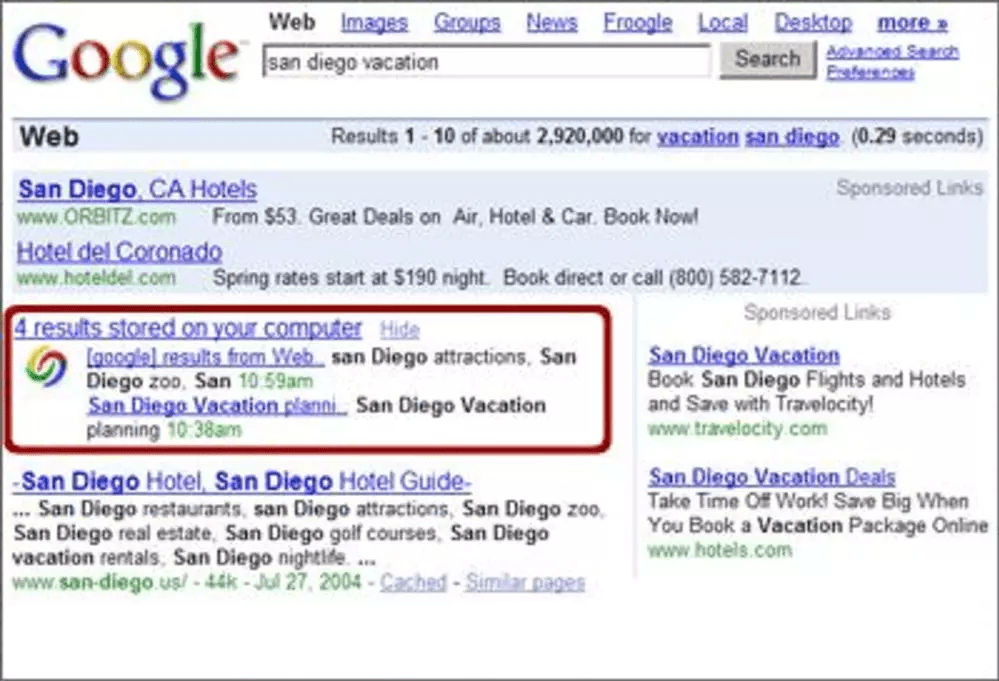In the image, a Google search results page is displayed prominently. At the top of the page, the iconic Google logo is visible, immediately recognizable with its distinct color scheme. Below the logo, several search categories are listed, including Web, Images, Groups, News, Froogle, Local, Desktop, and an option for More.

The search query has returned a variety of results. Under the Web category, specific results are shown, such as "San Diego, California hotels," "San Diego vacation," and "San Diego vacation deals." Additionally, there are four results stored on the user's computer related to the search. Each result is accompanied by a brief snippet of information, helping the user quickly identify the most relevant links. This image captures a typical user's interaction with Google's search engine, showcasing its broad range of categories and the efficiency in delivering search results.